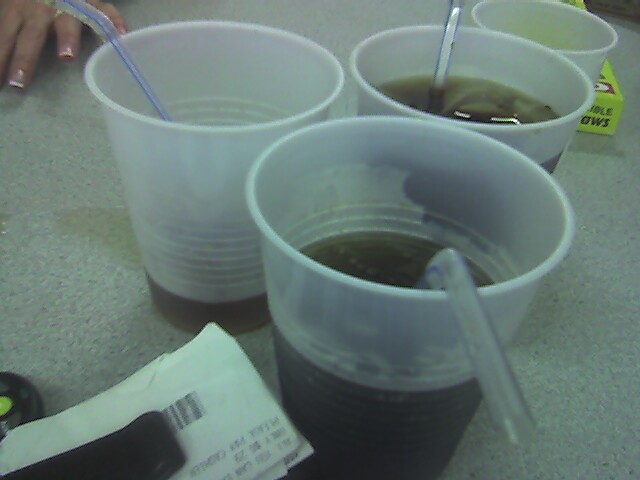This photograph, taken indoors, showcases a light gray speckled table laden with four opaque plastic disposable cups, each containing varying levels of a dark brown, bubbly liquid—likely a soda. The cups are equipped with clear bendable straws featuring blue stripes. In addition to the cups, the table holds a box labeled "bendable straws," revealing the origin of the straws. Scattered nearby are a stack of envelopes, a set of car keys with a beeper, and a partially obscured receipt—suggesting an informal setting. The top left corner of the image prominently features a woman's hand with a French manicure, delicately resting on the table.